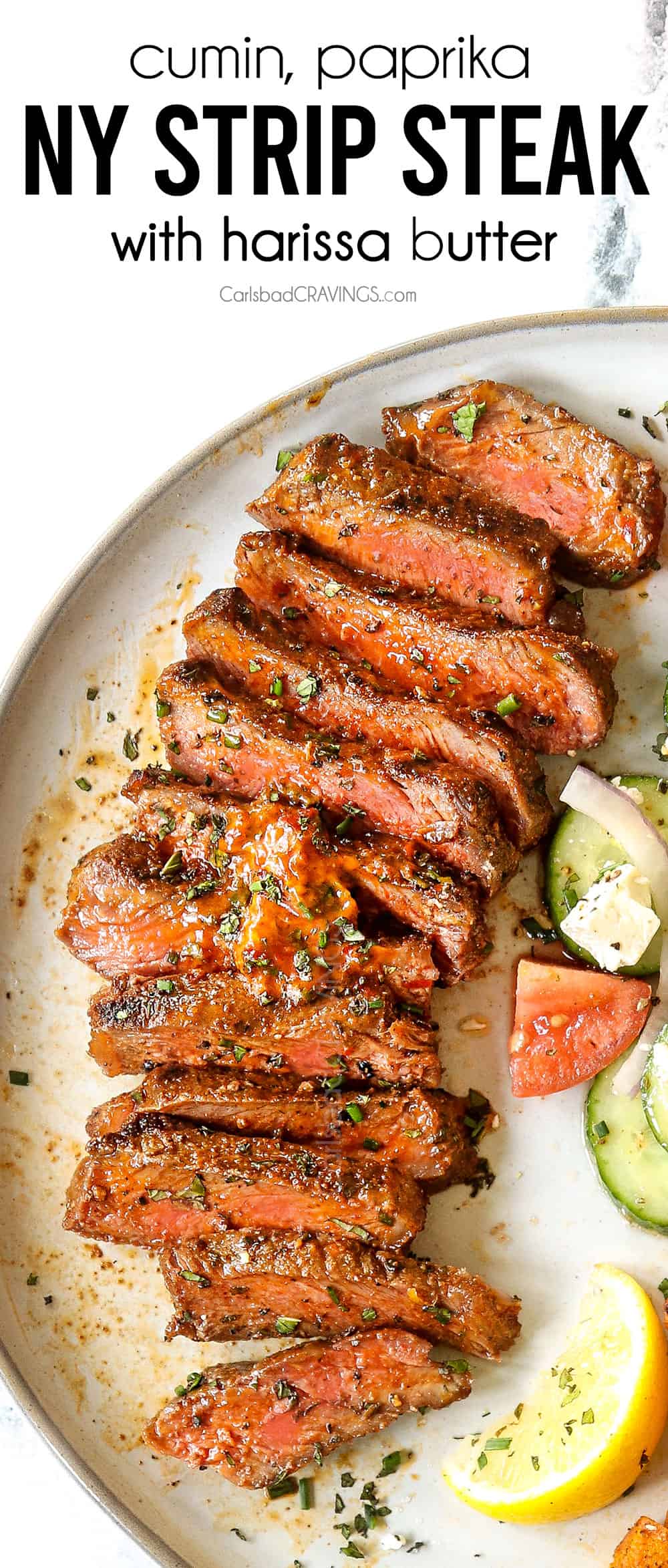The image is an advertisement for a steak recipe displayed as a front image of the recipe. At the top, the text reads "Cumin Paprika New York Strip Steak with Harissa Butter" and below it, in smaller font, is the website "carlsbadcravings.com". The centerpiece of the image is a whitish plate holding the cumin and paprika-seasoned New York strip steak, cut into thin horizontal strips that are cooked to medium-rare, with a reddish-brown hue and a slightly pink center. The steak is garnished with various herbs and spices, with harissa butter in the middle, exhibiting a dark orange color. Accompanying the steak on the plate are sliced cucumbers, tomatoes, a lemon wedge, and some onions, all carefully arranged beside the main dish.